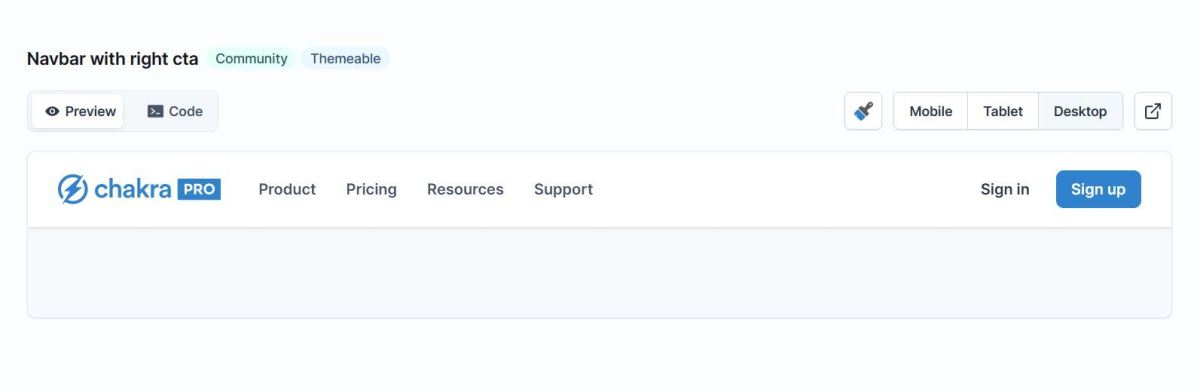**Detailed Descriptive Caption:**

The screenshot showcases a rectangular interface that is wider than it is tall. At the top-left corner, there is a navigation bar featuring a call-to-action button aligned to the right. The navigation bar includes the word "Community" in black lettering against a light teal background. Adjacent to "Community," the word "Themable" is displayed in blue with a light blue background exclusively surrounding it.

Below this, there's a toggle button designed as a rounded rectangle with a gray border and a lighter gray background. This toggle features a white button labeled "Preview" accompanied by an 'eye' symbol to its left. To the right of "Preview," there's a button labeled "Code," which includes a right-arrow symbol that looks like an underscore within a square with rounded corners, rendered in black.

Further to the right, a set of icons represent different functionalities: a paintbrush icon, symbols for mobile, tablet, and desktop devices, and an icon perhaps representing a send link. Below these is a lightning bolt encircled, followed by the text "Chakra Pro."

The menu options include "Product," "Pricing," "Resources," and "Support." Towards the far-right of the interface, there are options to "Sign In" and "Sign Up." The "Sign Up" button stands out with white lettering on a medium blue background.